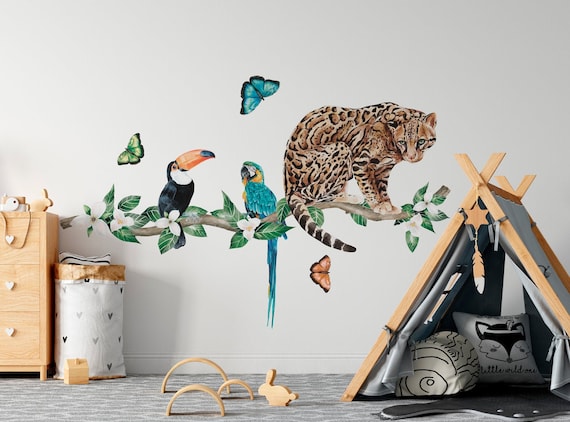The image portrays a meticulously staged children's bedroom, likely photographed for a home magazine or furniture advertisement. Dominating the scene is a pristine white wall featuring elaborate, painterly wallpaper—a horizontal tree branch adorned with intricately detailed wildlife. Perched on the branch are a bobcat, a toucan, a bird with an exceptionally large beak, and a striking blue bird boasting long tail feathers. The vivid, nature-inspired tableau is further animated by three butterflies flitting above and below the branch. 

On the right side of the image rests an A-frame wooden teepee with no front or back panels, inside which lie two plush cushions for a child to recline on. The teepee is whimsically embellished with a hanging feather and star, as well as a playful cartoon cutout of a cat. To the left corner, a small wooden dresser with heart-shaped drawer pulls stands next to a round laundry basket. On the carpeted floor in front of the scene are a wooden cutout of a bunny rabbit and three rainbow figurines in varying sizes.

The image strikes a harmonious balance between functional furniture and enchanting decor, vividly capturing the essence of a child's imaginative sanctuary.